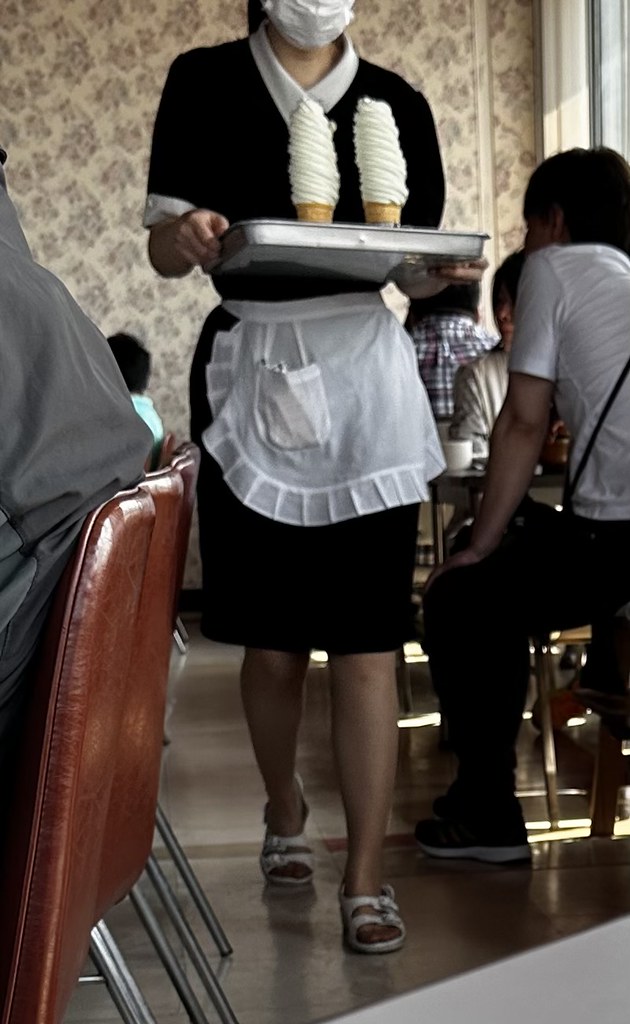This colored photograph, taken indoors during the daytime, captures a scene inside a quaint restaurant with sunlight streaming through a window on the upper right. The back wall features an unattractive brown and red floral wallpaper. On either side of the restaurant aisle, people are seated on leather-backed, rather cheap-looking brown chairs. You can’t make out any faces clearly, but there are some details evident: a man in a light t-shirt with a younger child on one side, and a man in a gray shirt with another person in a greenish shirt on the other.

Centered in the image is a waitress in motion. She's wearing white sandals, and a standard black uniform akin to a maid's, complete with a short-sleeved dress, a white collar, and a ruffled white apron. Concerned about COVID-19, she has a white mask covering her face. She balances a silver tray holding two towering, soft-serve vanilla ice cream cones. The overall atmosphere hints at a casual and somewhat outdated setting, augmented by the wallpaper and simple furnishing.